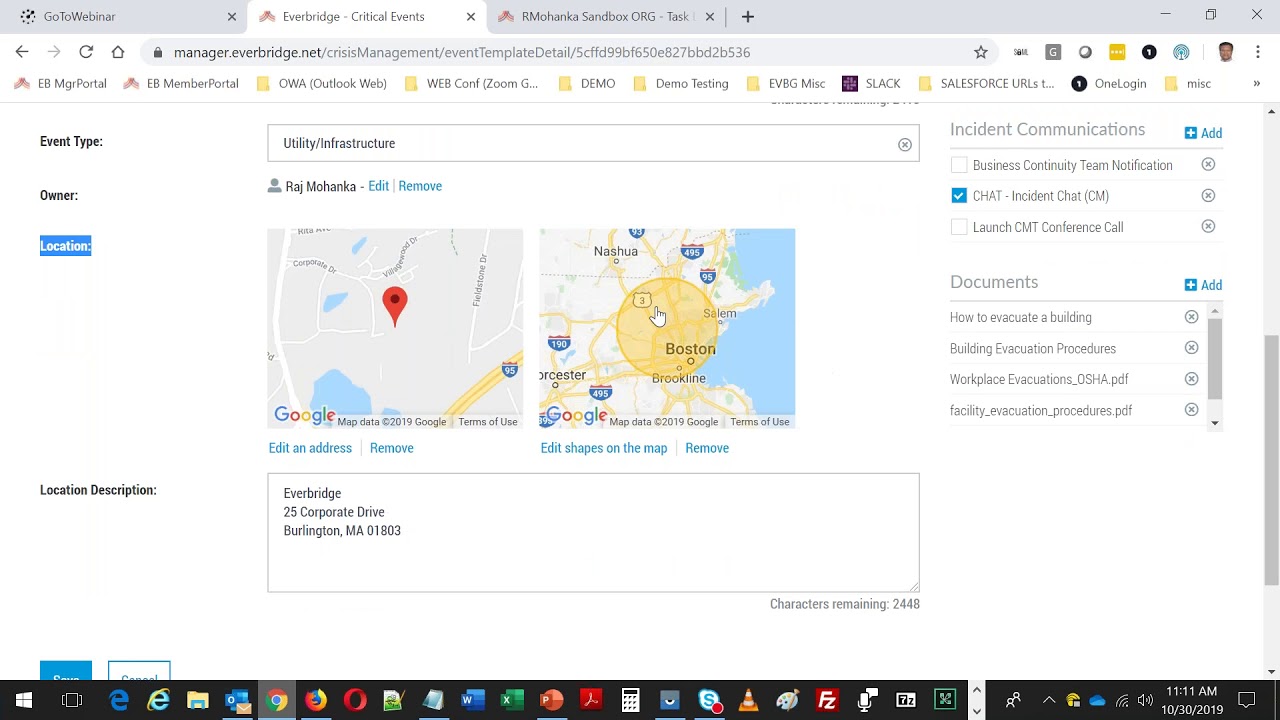Screenshot Description: 

The screenshot showcases an open web browser with visible elements organized in a detailed layout. 

- **Browser Tabs:** Along the top, there are three tabs visible against a grey background. The second tab is highlighted in white, indicating it is the currently active tab.

- **URL Bar:** The navigation bar at the top displays the URL: "manager.everbridge.net."

- **Website Layout:**
  - **Background:** The webpage background is white.
  - **Left-Hand Column:** 
    - **Headings:** In bold, the first heading reads "Event Type," followed by some spacing. Next, the heading "Owner" appears, again followed by a space. Below it, the highlighted heading "Location" is displayed, indicating the user's current focus. Near the bottom, the title "Location Description" is present.
    - **Fields and Content:**
        - **Event Type:** Next to this label, there is a text box containing the text "Utility Infrastructure."
        - **Owner:** This section includes an icon depicting a person's head and shoulders, alongside the name "Raj Mahanka." Options to edit or remove this name are visible.
        - **Location:** This section shows two maps from Google Maps, with editing or removing options available for the displayed address.
        - **Location Description:** The text "Event Bridge 25 Corporate Drive, Burlington, MA 01803" is provided.

- **Right-Hand Side Panel:**
  - **Information and Controls:** Additional information is present here, with a scroll bar indicating more content below.
  - **Incident Communications:** Listed beneath this heading, there are three options, one of which is checked for "Chat."
  - **Documents:** A list of four documents is displayed in this section. 

The screenshot offers a detailed visual overview of the Everbridge Manager interface, with navigation controls and clearly defined sections and fields.